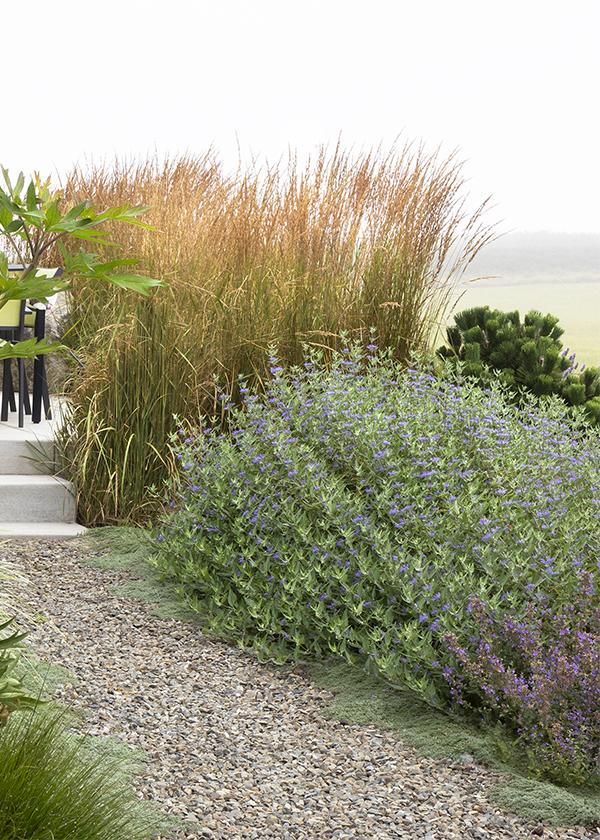The image depicts a gravel walkway composed of small, flattened rocks, bordered by various plant species. On the left side, tall grasses and weeds partially encroach upon the path, with a branch of a tree visible in the upper left corner. The right side features a large bush adorned with blue and purple flowers, dominating the foreground. Behind this bush, very tall grass transitions from green at the base to dark orange-brown at the tips. The background is blurred but reveals a body of water with mountains in the distance. Additionally, a portion of the walkway appears to lead up to two or three concrete steps, adjacent to what might be patio furniture legs. This suggests the scene could be coastal or desert, given the tall beach grass and potential succulent plants. Touches of blue and cream color further enhance the backdrop, likely indicative of the sky and sand.